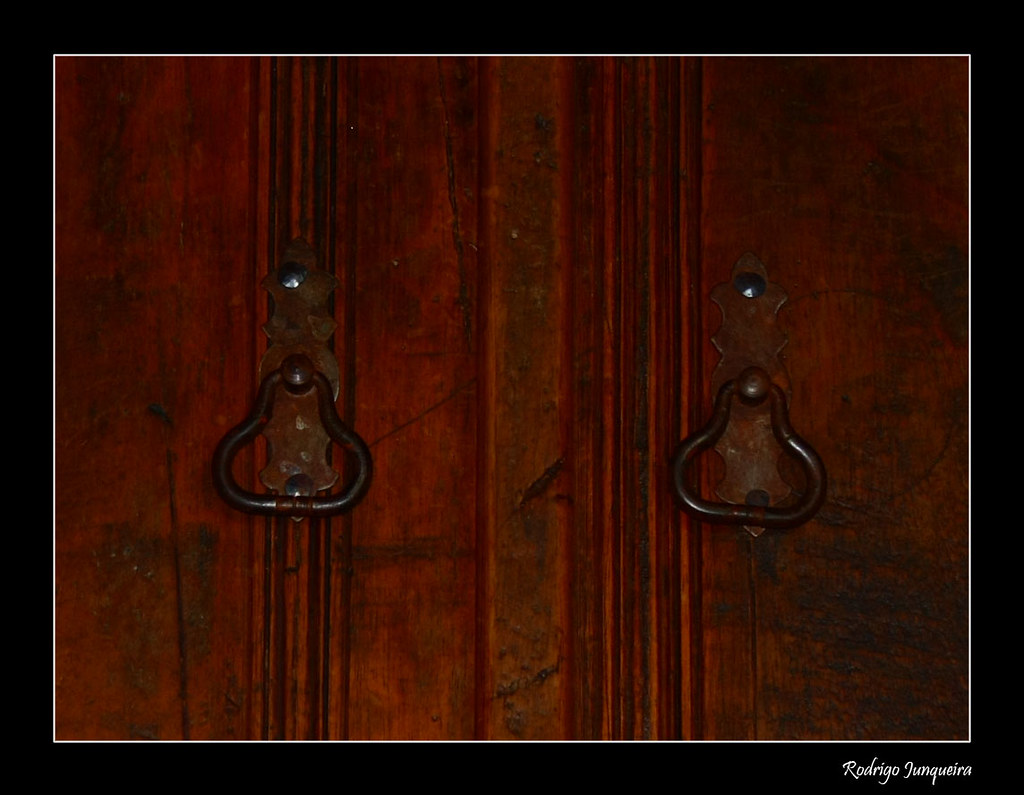The image showcases a close-up, side view of a wooden panel stained in a dark, cherry-red color with striations running vertically across its surface. Encased within a double border—a thin white inner line and a thicker black outer frame—the panel features two ornate, vintage-looking handles positioned symmetrically about two inches from each edge. Each handle consists of a small, flat metal plate fastened with steel pins, and a hoop-like piece of wire in the center, reminiscent of antique cabinet pulls. The handles appear dark and tarnished, adding to the antique aesthetic. In the bottom right corner, the black border contains the name "Rodrigo Juanqueria" in white lettering, lending a personalized touch to the image.